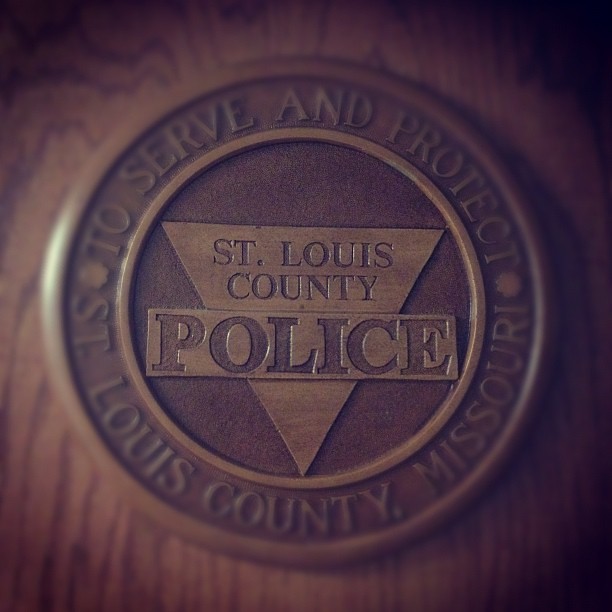The image shows a circular medallion, copper-colored in appearance with gradients of lighter brown tones, mounted on a wooden background. The outer edge of the medallion features etched, all-caps text that reads "TO SERVE AND PROTECT" at the top and "ST. LOUIS COUNTY, MISSOURI" at the bottom. Inside the medallion, there is an engraved upside-down triangle, within which the words "ST. LOUIS COUNTY" are inscribed at the top. Across the middle of the triangle, a rectangle with the word "POLICE" is prominently displayed. The background and edges of the image are slightly blurry, with blacked-out corners, enhancing the central focus on the medallion and giving it a distinct, mounted plaque-like appearance.